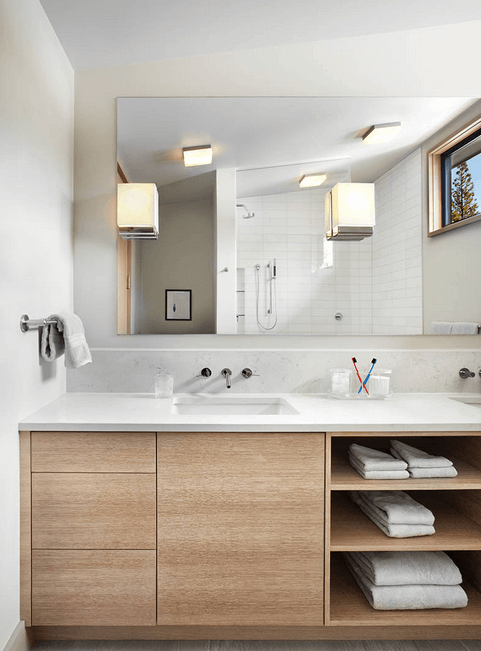This photograph captures an elegant bathroom bathed in daytime light, reflecting a serene and tranquil ambiance. The light streaming from outside subtly illuminates the scene, and through the mirror's reflection, a glimpse of a tall, verdant tree bathed in the soft glow of a setting sun is visible. The sky outside exhibits a gradient of blue hues, transitioning from a darker to a lighter shade due to the sunset.

At the bottom center of the frame, a pristine sink with gleaming silver knobs stands out, with a set of intricately placed cabinets below and to the sides. The cabinet setup includes three compartments on the left, a central cabinet, and additional storage on the bottom right, which neatly holds a collection of towels—a pair on the top shelf, one in the middle, and another at the bottom.

To the left of the sink, a white washcloth is carefully draped over a silver rack, adding a touch of softness to the room's clean lines. On the right side of the sink, two toothbrushes, one red and one blue, are crossed in an x-formation, hinting at a personal touch.

The room is well-lit by a large square light fixture on the ceiling, complemented by additional lighting around the mirrors, ensuring a bright and inviting environment. The bathroom's design also includes a shower area, partially visible, featuring a sleek showerhead with an adjustable extension for flexible use.

This detailed composition highlights both the functional and aesthetic elements of the bathroom, offering a glimpse into both the indoors and the serene natural scenery outside.